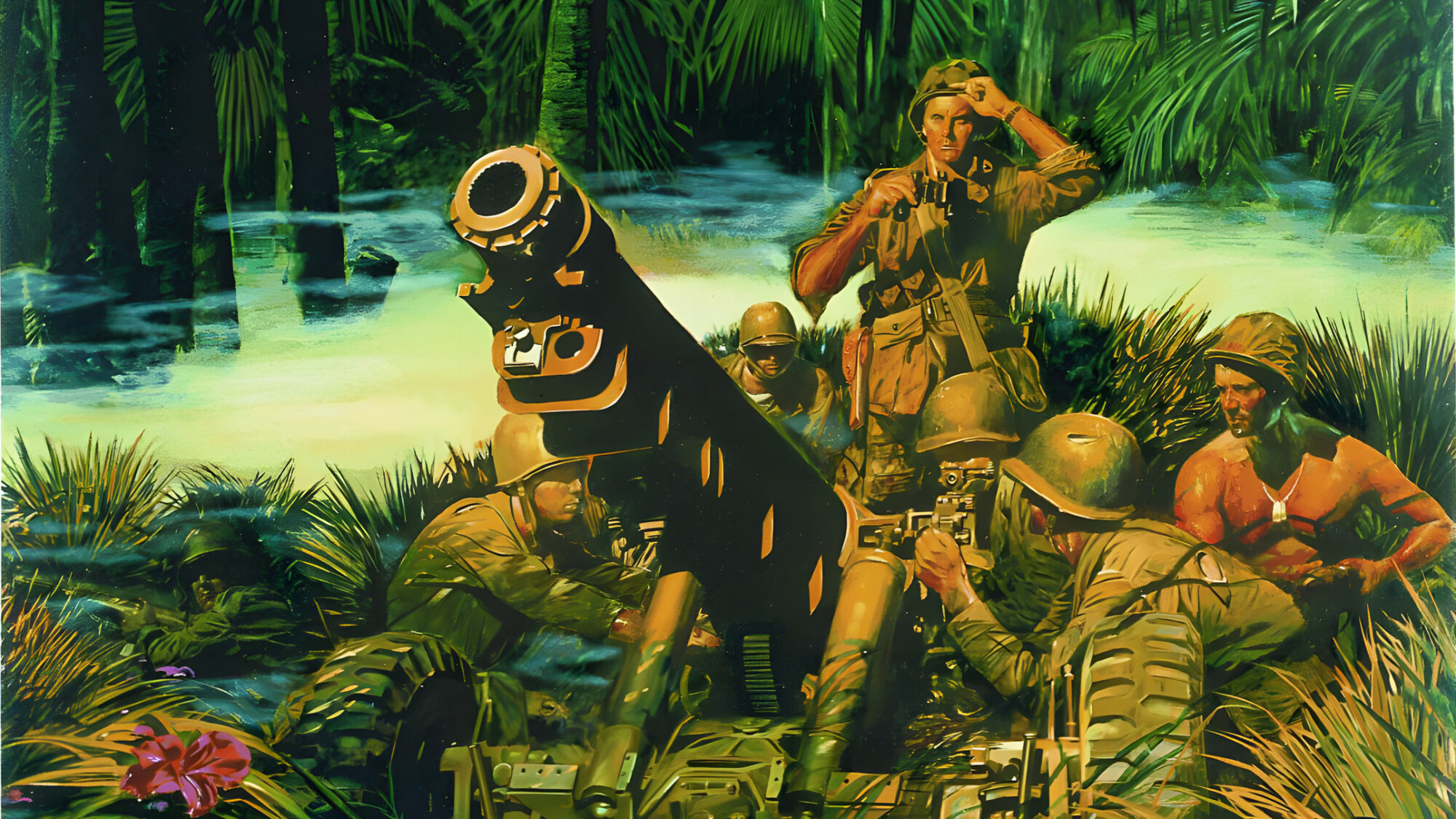The illustration depicts a crew of U.S. soldiers in World War II, situated in a swampy, Southeast Asian locale, characterized by an array of lush greenery, palm fronds, and a body of water in the background. The soldiers, clad in drab olive green uniforms, are centered around a large artillery piece, most likely a howitzer, with a long, wide-barreled cannon mounted on thick rubber treads. Among the crew, four soldiers are diligently setting up the howitzer, preparing it for what appears to be a lobbing operation. One soldier stands out, shirtless with dog tags dangling against his chest, possibly marked by a green bandana around his neck. Meanwhile, a commanding figure, distinguished by a different helmet which could imply Marine affiliation, stands upright and adjusts his binoculars, likely assessing their targeting accuracy. The scene is bathed in a slightly washed-out palette, enhancing the raw, harsh atmosphere of their environment. The rich detail includes features like hydraulic pumps connecting the gun to its harness and a singular pink flower blooming amidst green grass in the bottom left, adding a contrasting touch of life and color to the somber tensions of wartime.